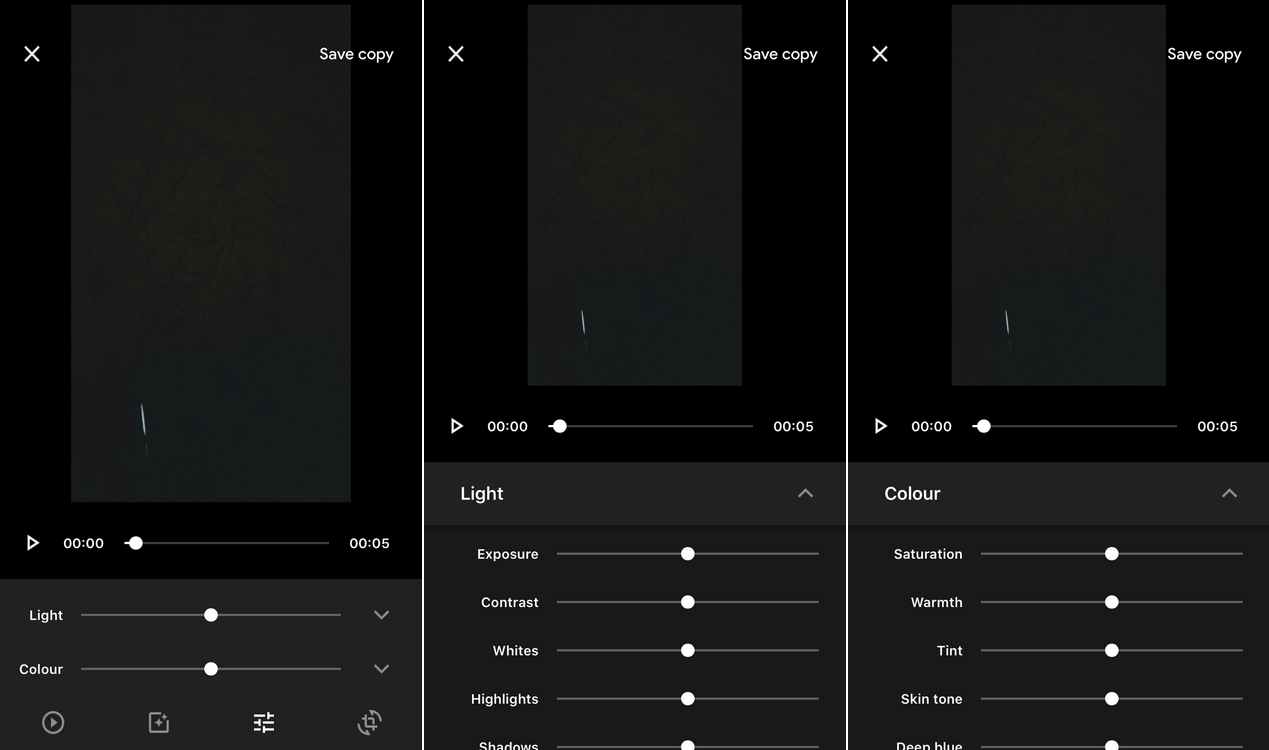The image is composed of three different phone screenshots arranged side by side: one on the left, one in the center, and one on the right. Each screenshot features a predominantly black background with an audio player at the top, where the playback bar is paused at the five-second mark. In the upper-right corner of each screenshot, a "Save Copy" button is visible, while on the upper-left, an "X" button for exiting the page is present. 

The audio player, prominently positioned in the upper-middle region of each screenshot, shows a play button with a timestamp of "00:00" on the left end of the progress bar, which clearly indicates a position of 5 seconds by showing "00:05" on the right end. Beneath the audio player, two drop-down menus labeled "Light" and "Color" are displayed.

In the first screenshot, only the drop-down menus are visible, not expanded. In the center screenshot, the "Light" drop-down menu has been selected, revealing its options: Exposure, Contrast, Whites, Highlights, and Shadows. The right screenshot shows the "Color" drop-down menu in its expanded state, displaying options such as Saturation, Warmth, Tint, Skin Tone, and Deep Blue.

Overall, these screenshots provide a clear, step-by-step depiction of the audio editing interface on a mobile device, including specific functionalities and options within the "Light" and "Color" settings.